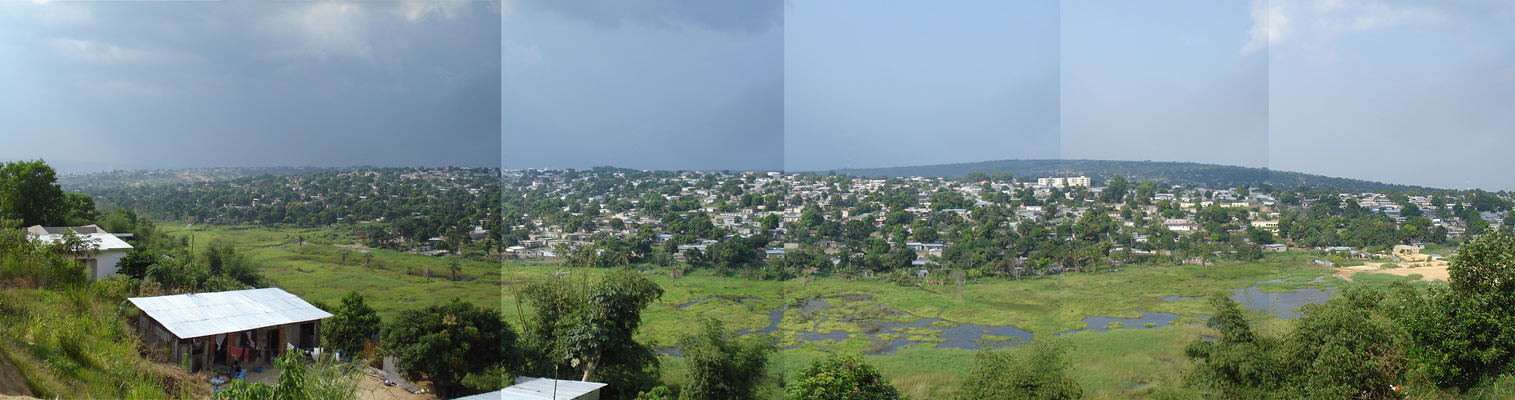This detailed panoramic image captures a vibrant tropical town nestled in a marshy valley environment, presented in landscape orientation. The image, composed of multiple sections stitched together to create a smooth mural effect, is longer than it is tall. At the bottom left corner, there are small structures with corrugated metal rooftops, surrounded by clutter and clothes. The foreground features a lush green marshland with water and vegetative growth, transitioning to a beach on the right-hand side. The village, predominantly composed of white and beige single-story houses and a few three to four-story concrete buildings, sprawls across a gentle hill. In the background, a large cityscape stretches across the horizon beneath an overcast sky, with visible patches of blue sky and distant rainfall, creating a dynamic weather contrast. The entire scene appears slightly folded due to the creases in the poster from which the image is taken, adding to its textured realism.